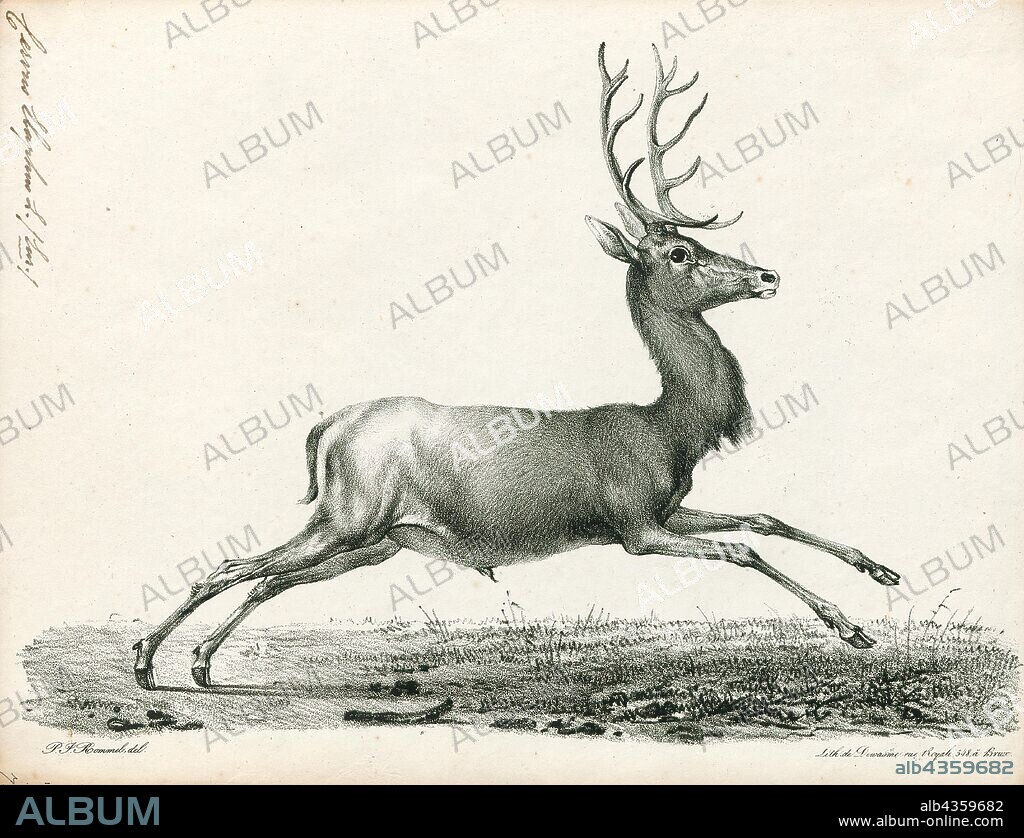A detailed black-and-white, vintage illustration of a male deer in profile forms the focal point of this landscape-oriented image. The deer, depicted in mid-trot with both front legs raised and its long hind legs firmly on the ground, has a large rack of antlers and is sketched in varying shades of gray. The ground beneath the deer shows a rendition of parched, grassy patches and rocks, contributing to a rustic wildlife setting. The off-yellow, off-white background is overlaid with a diagonal watermark repeatedly displaying the word "ALBUM" in gray capitals. The top left corner features a barely legible, black cursive signature turned on its side, with additional illegible signatures on the bottom left and right corners. Dominating the bottom of the image is a black rectangular bar, with the left side displaying "ALBUM" in gray, capital letters and the right side featuring an alphanumeric code, "ALB 4359682," followed by the URL "www.album-online.com," both in white text. The overall composite utilizes a limited color palette of gray, off-yellow, and off-white, emphasizing its vintage, monochromatic style.